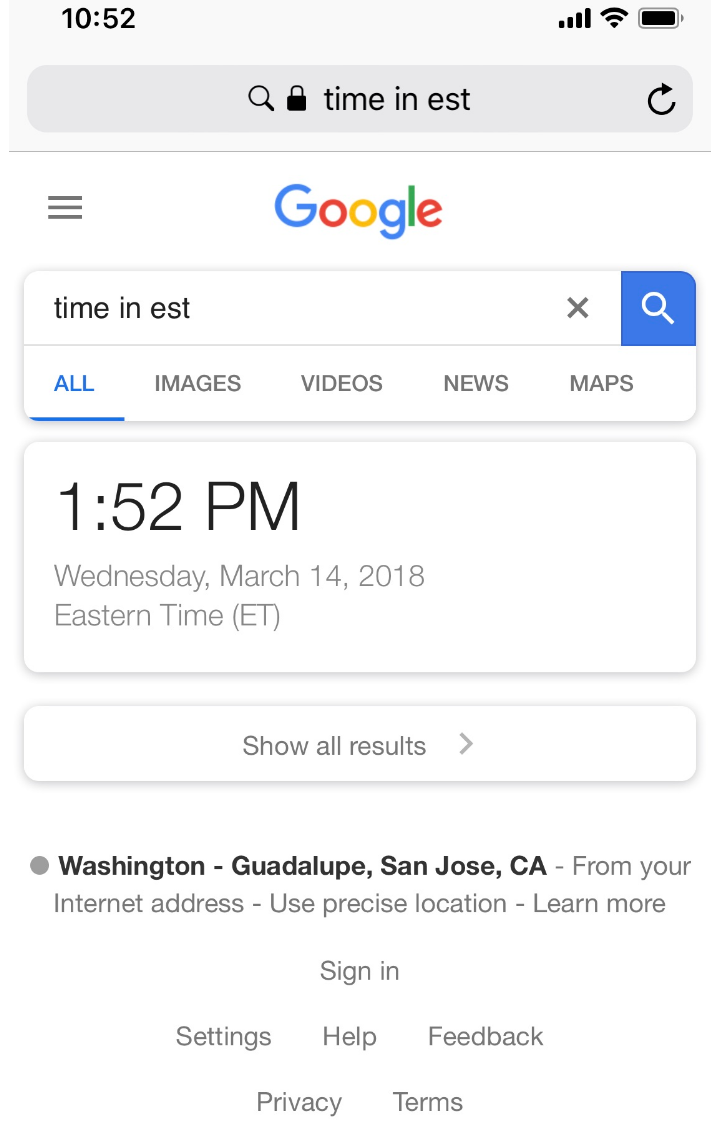Detailed Caption: 

The image depicts a screenshot taken from a smartphone, oriented in a portrait rectangle format. At the very top of the screen, the time is displayed as "10:52" in bold digits. The status bar includes icons indicating full Wi-Fi signal strength with four bars, a Wi-Fi symbol, and a fully charged battery.

Below the status bar, there is a shaded-in area featuring a magnifying glass icon and a lock symbol, with "Time in EST" noted next to it. An arrow icon suggests navigation to the previous screen. 

The next section showcases a clean white space with three horizontal lines (likely a menu icon) followed by the vibrant, colorful Google logo centered on the screen. Below this, again on a white space, "Time in EST" is repeated alongside a small “X” on the right, presumably for dismissing a search result or prompt. A blue magnifying glass icon appears next to this.

The following line highlights "All" in blue text, indicating the currently selected search category. Other available options such as "Images," "Videos," "News," and "Maps" follow in grey text. 

Below these options, the time "1:52 PM" is stated, accompanied by lighter printed text reading "Wednesday, March 14, 2018, Eastern Time," and the abbreviation "ET" stands out in capital letters. 

Further down, an option labeled "Show all results" is presented, followed by a geographical reference: "Washington to Guadalupe, San Jose, CA," attributed to the user’s internet address. This is followed by an option to "Use precise location - Learn more."

At the bottom of the screen, there are additional links: "Sign in," followed by "Settings," "Help," and "Feedback." The very bottom includes legal links: "Privacy" and "Terms," each separated by a space.